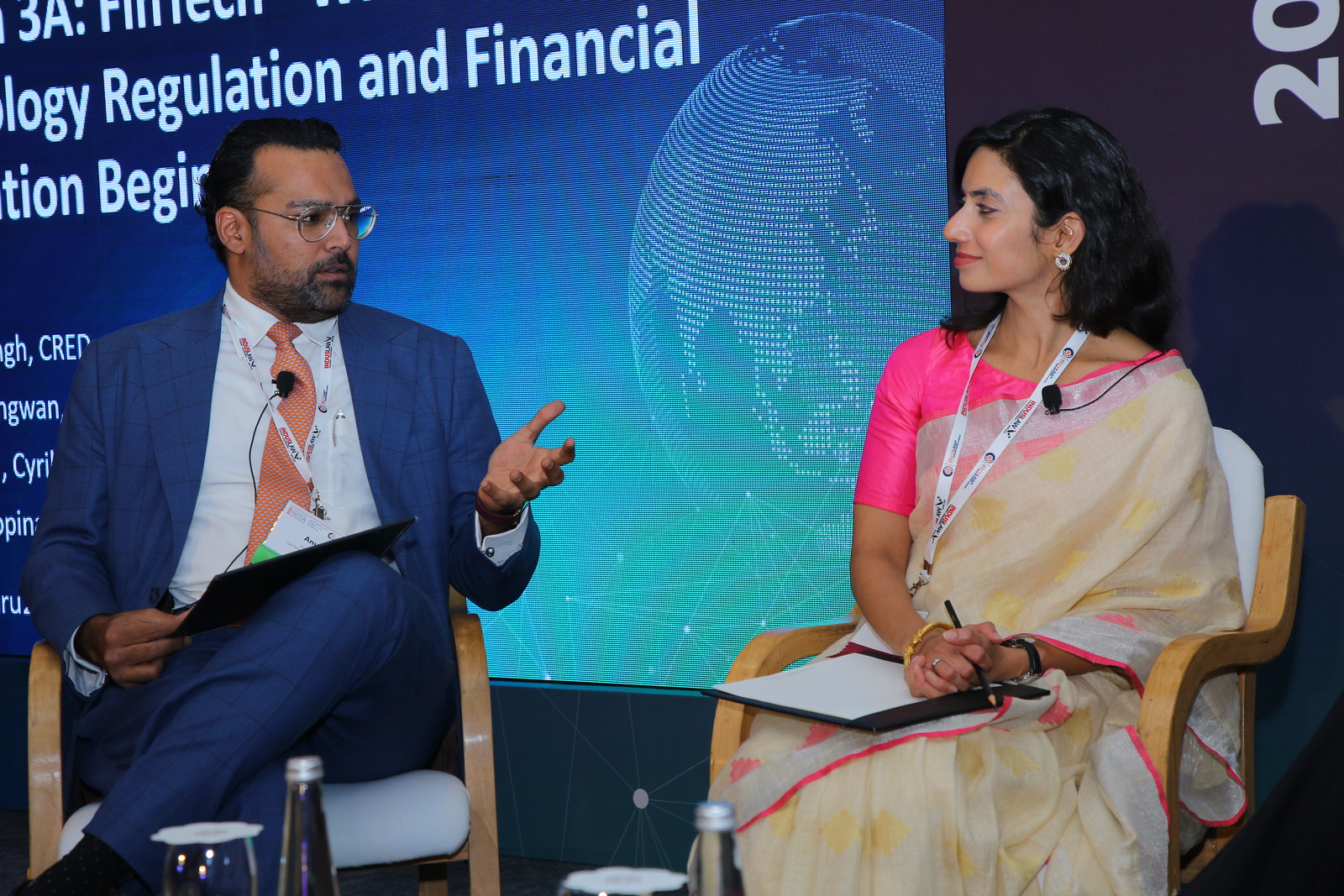The photograph, in landscape orientation, depicts two individuals engaged in conversation, seated on a podium at what appears to be a convention or event. The man on the left wears a dark blue suit, white shirt, and an orange tie. He has dark hair, dark skin, a beard, and wire-rimmed glasses. A white lanyard hangs around his neck, and he gestures with his left hand while speaking. The woman on the right, who appears to be South Asian, wears a pink shirt with a beige sari draped over her shoulder. She holds a clipboard with a piece of paper and a pencil in her lap, her hands clasped. She also has a white lanyard and a speaker microphone atop her robe. In front of them are bottles of water and cups resting on a table. The background features a projection screen displaying a partial image of a globe with fragmented white text at the top, including partially visible words like "3A, L-O-G-Y Regulation and Financial, T-I-O-N-B-E-G-I," and random letters "G-H-C-R-E-D-C-Y-R," along with the number "20" in the top right corner. The photograph, likely captured from a TV screen, exudes a formal and academic ambiance.